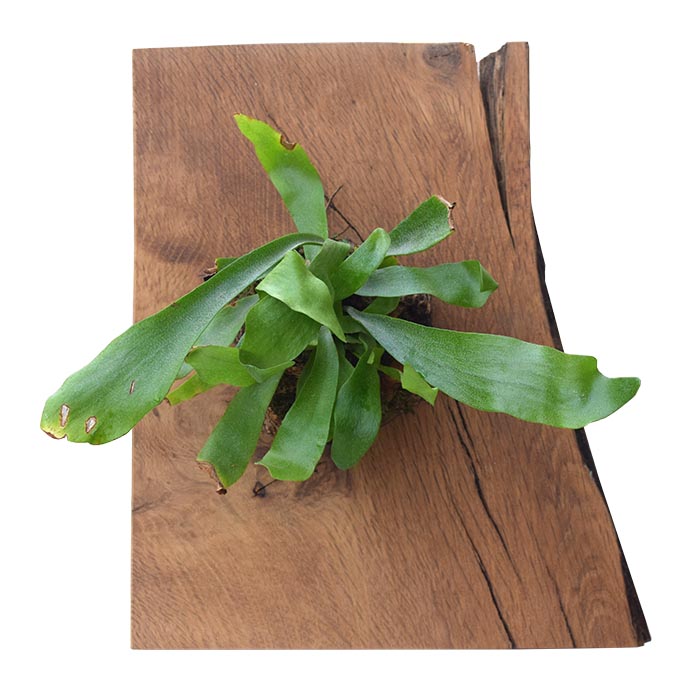This color photograph depicts a partially cropped slab of wood with a natural grain, showcasing intricate cracks and seams throughout its surface. Emerging from a central knot in the wood is a staghorn fern, notable for its long, thin fronds. The fern has approximately ten leaves radiating in various directions—upwards, downwards, and to the sides. The leaves are narrow, somewhat intertwined, and possess a waxy texture. While primarily fresh and green, some leaves exhibit notable imperfections: small holes and browning at the edges and tips. The wood, likely cut at a right angle, rests against a white or transparent background, further highlighting the green vibrancy of the plant against the rustic texture of the wooden slab.